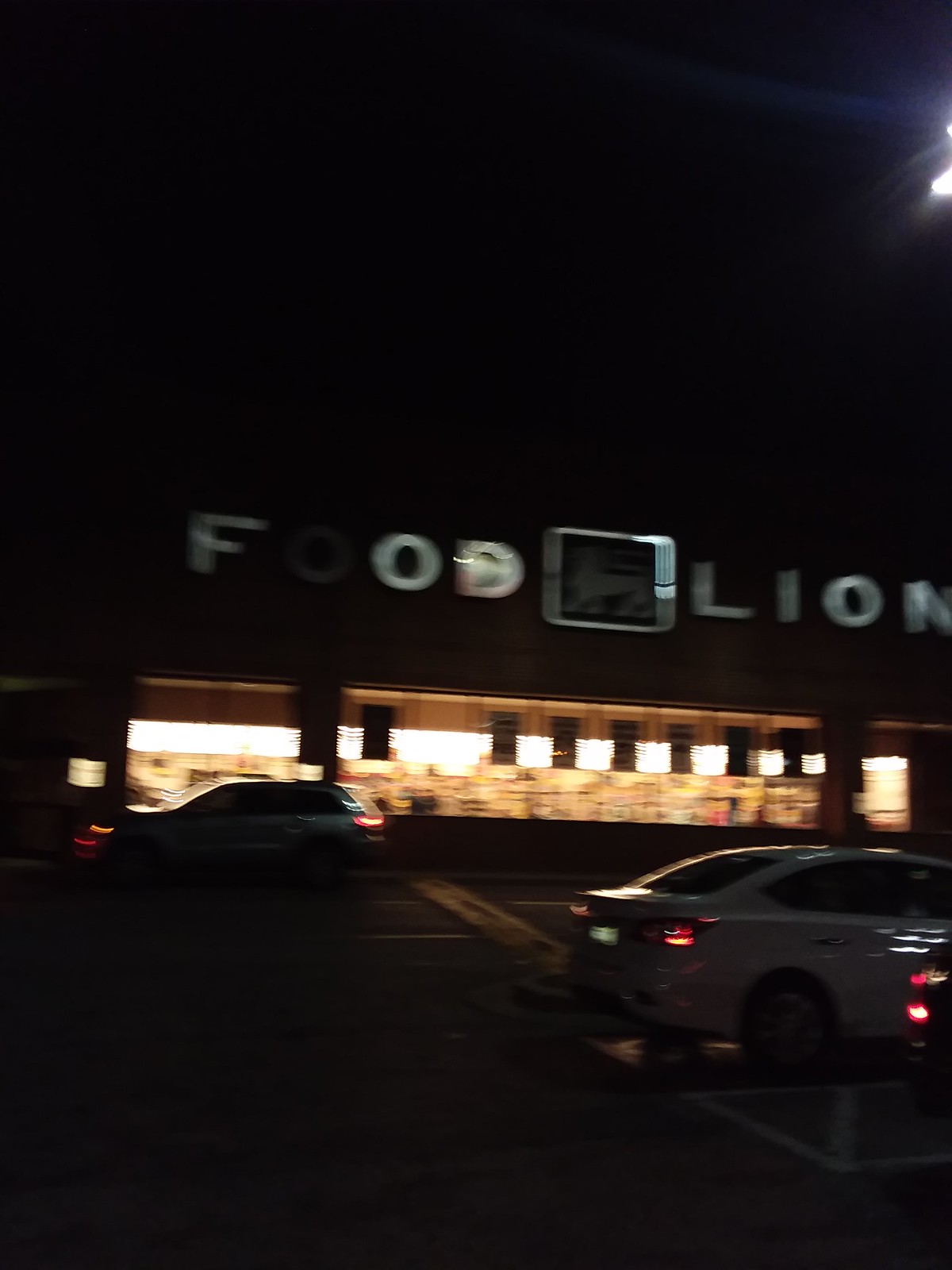This photograph, taken at night, captures a Food Lion grocery store from the vantage of its parking lot. The illuminated sign atop the building prominently displays the store's name, though the 'O' in 'Food' is burnt out, lending a distinctive look. Adjacent to the sign, a small rectangular box with a glowing lion logo can be seen. Despite the overall blurriness of the image, likely due to the nighttime setting, the scene is detailed with small yet telling elements. 

The single-story building has lights on inside and shelves of items are faintly visible through the windows, suggesting an active store. Outside, three cars are situated in the parking lot. A white car with its lights on is parked facing to the right, next to a darker vehicle whose rear end is partially visible. Additionally, a white or silver sedan with its lights on is parked close to the building, facing left. The scene is framed by a streetlight in the top right-hand corner, casting illumination onto the otherwise dry and dimly lit parking lot. The overall composition captures the mundane yet specific details of a nighttime visit to a grocery store.